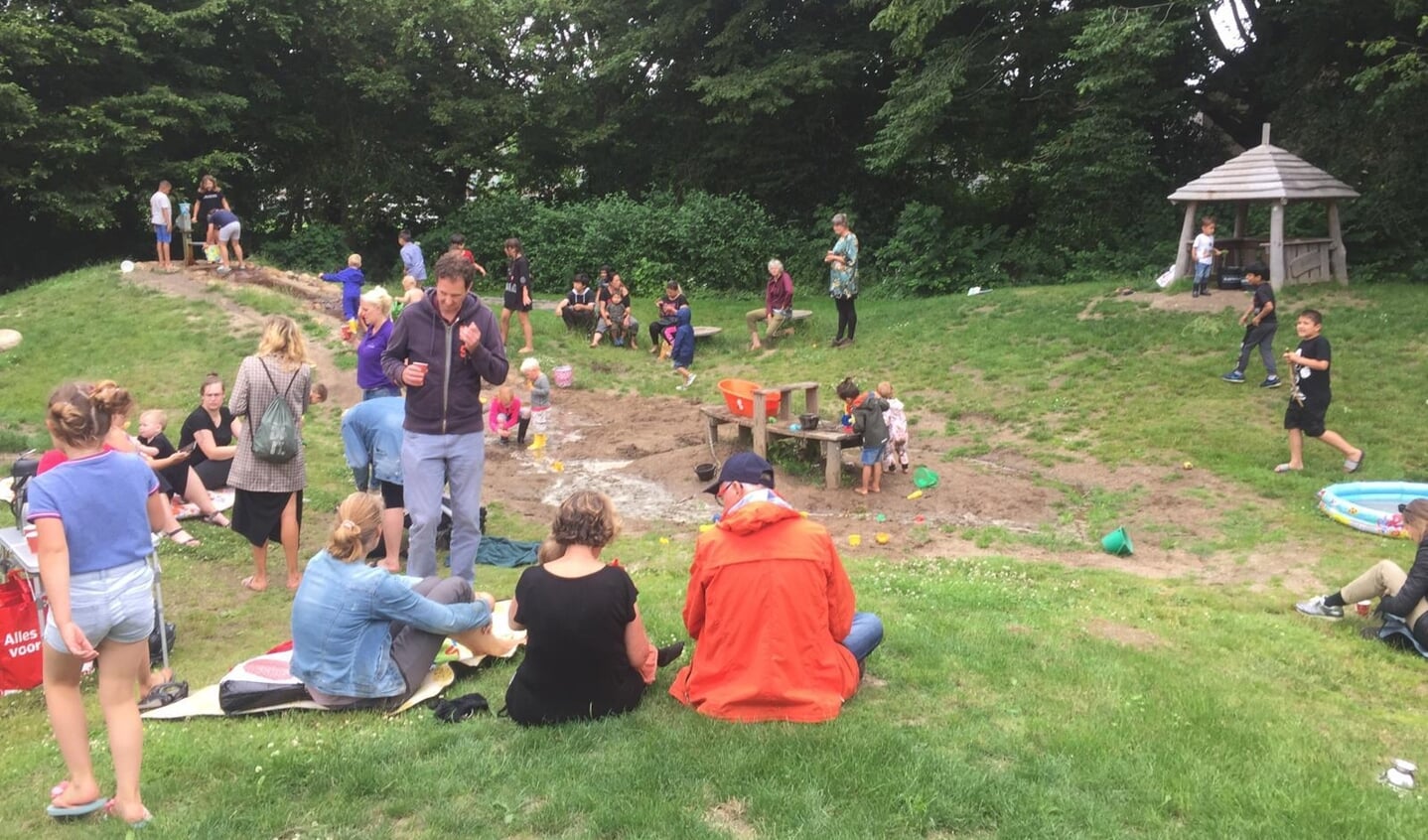The image depicts a lively park scene with a large group of people of all ages spread across a grassy and hilly area. In the foreground, a young girl wearing a purple shirt and jean shorts walks on the bottom left, while three people nearby are seated on the grass, engaged in a conversation with a man in jeans and a dark hoodie. At the center of the scene, children enthusiastically play in a sandpit, constructing sandcastles and other structures. Nearby, on the center right, there's a kiddie pool attracting more kids. The upper right features a wooden picnic table under a hut, and in the background, dense dark green trees frame the event, stretching across the horizon. To the left, a slightly elevated area features a trail where people can be seen setting up activities amidst the dirt. People are scattered throughout the park, some sitting on blankets with their belongings, others exploring the different play stations. The park’s landscape is undulating, creating a dynamic setting of small hills and valleys that add to the charm of the event.